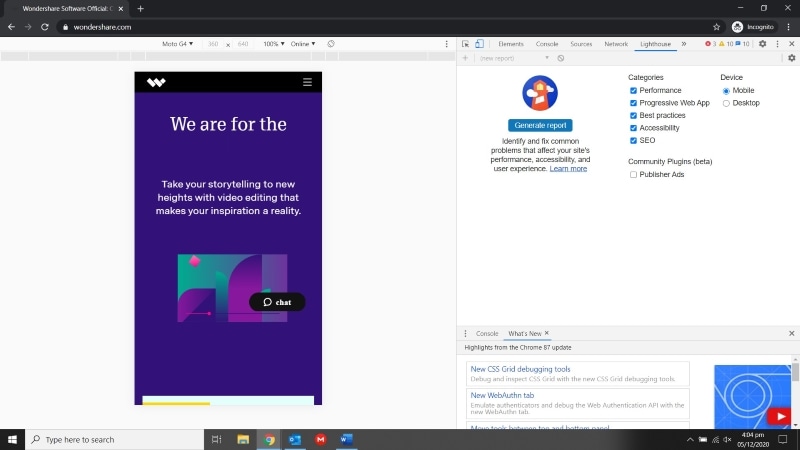The screenshot depicts a webpage from Wondershare, an online software office. The resolution of the image is quite poor, but some key details can be discerned. The URL at the top reads wondershare.com, and you are currently on a tab labeled "Wondershare Software Office."  

On the left side of the page, there is a banner with blue-purple background displaying a motivational message: "Take your storytelling to the next height with video editing that makes your inspiration a reality." Below this message, an image of a cell phone is shown. 

Towards the bottom left side, there is a black chat button with white text. On the right side, there is another section that details site performance features: "Create report, identify and fix common problems that affect your site's performance, accessibility, and user experience." There is also a "Learn more" link in blue, underlined text, with the rest of the information in black.

Below this section, there are several categories listed: Performance, Progressive Web App (PWA), Best Practices, Accessibility, SEO, Device (Mobile and Desktop), Community, Plugins, Beta, Publish, and Ads. All these categories have blue check marks next to them, indicating selection, with a specific emphasis on the "Device" category showing mobile selected.

Above this content, a gray navigation bar is visible with the options: Elements, Console, Sources, Network, and Lighthouse. The current tab selected is "Lighthouse," which is part of the developer tools for auditing performance.